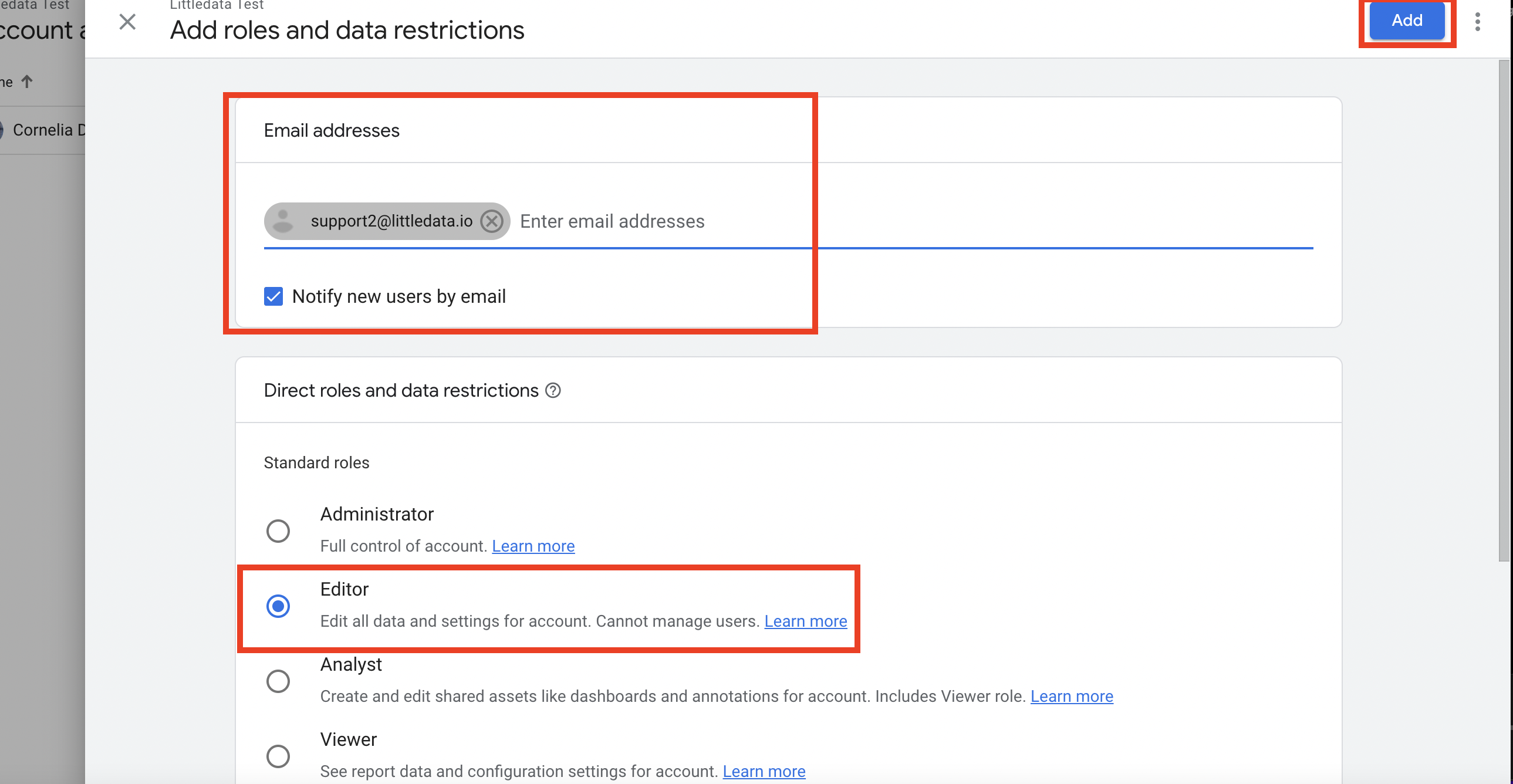Screenshot of a pop-up window for assigning roles and data restrictions 

The screenshot displays a pop-up window with a white header containing the text "Add Roles and Data Restrictions" in black. Within this header, a blue "Add" button with white text is prominently highlighted by a red rectangle.

The pop-up’s background is light gray, and the content is organized within white boxes. At the top, there is a section labeled "Email Addresses," which includes a field for entering email addresses and an option to "Notify new users by mail" with a checkbox. This entire section is surrounded by a red rectangle.

Below the email section, there is another content box titled "Direct Roles and Data Restrictions," listing four standard roles: Administrator, Editor, Analyst, and Viewer. The "Editor" role is selected (indicated by a blue radio button) and highlighted within a red rectangle, showing that the Editor role is currently selected.